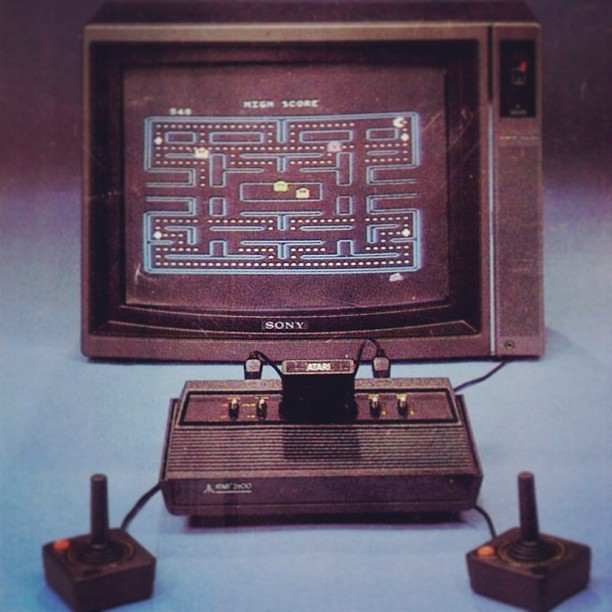The image depicts a vintage floor model tube TV with a silver border framing the screen on all sides. The TV is displaying a classic video game, namely Pac-Man. On the right side of the TV, there is a wider section that contains a black square at the top featuring black buttons with white lettering. Below this is a grilled section, presumably housing a speaker. At the bottom of this wider section, there is a 3.5mm jack port. In front of the TV, an Atari gaming system is visible, characterized by its black rectangular shape and an inserted Atari cartridge. Additionally, two joysticks are positioned on either side of the system, each featuring a red button and a tall cylindrical joystick in the center.